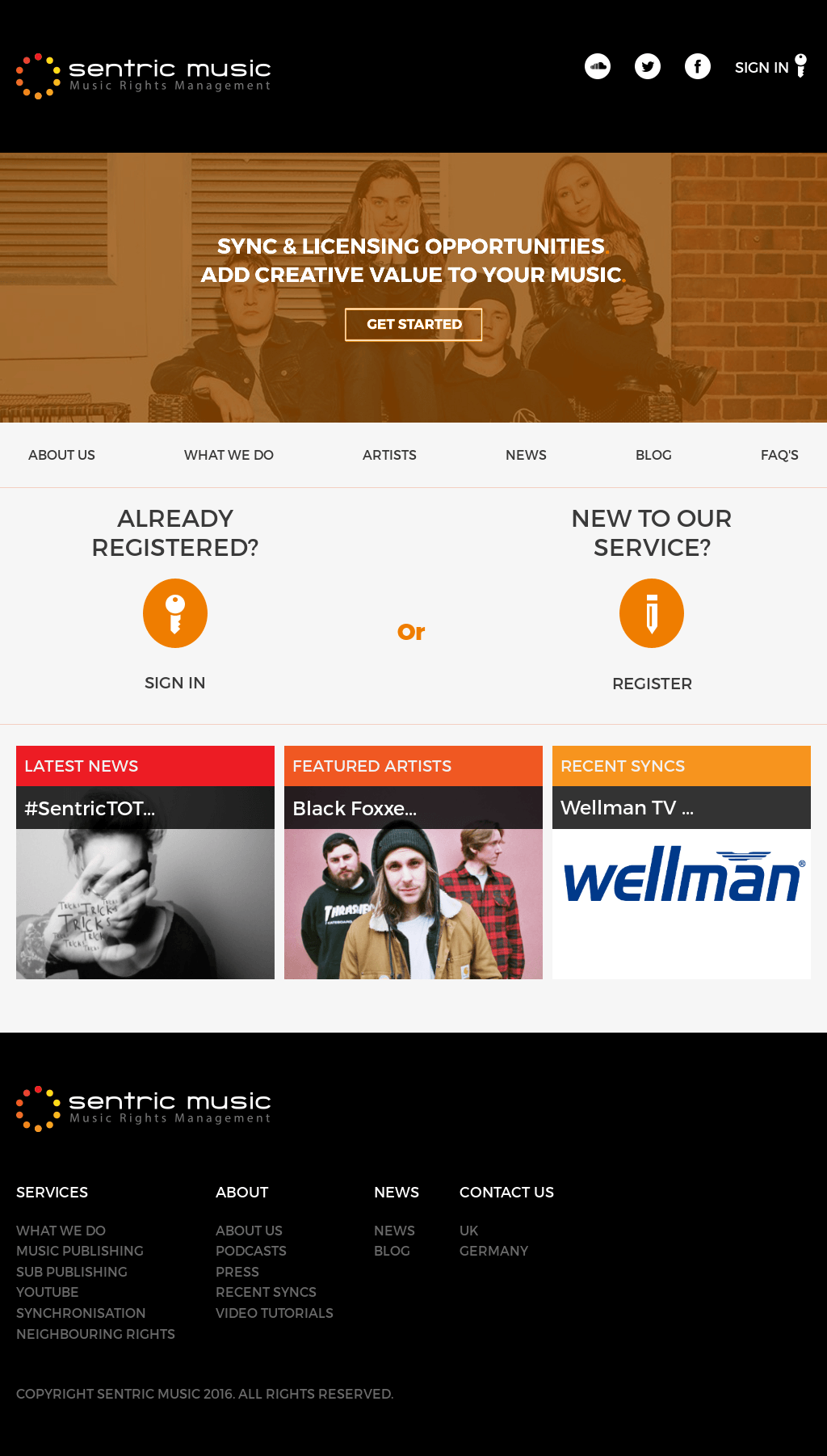The image is a vibrant and organized visual representation of the homepage for Centric Music Rights Management. On the left side, the Centric logo is prominently displayed - "S-E-N-T-R-I-C," with a creative design of concentric multi-colored circles in shades of orange, yellow, and red.

To the right of the logo, there are accessibility icons for social media platforms including SoundCloud, Facebook, and Twitter, complemented by a secure login icon represented by a lock, indicating the safety of the sign-in process.

Beneath the top header, there's an artistic orange watermark of a band in a casual setting: a man leaning against sound equipment, another with his hands on his face, a third sitting lower wearing a beanie, and a girl with her legs crossed looking towards the viewer.

Centrally, bold white text reads, "Sync and licensing opportunities, add creative value to your music," inviting users to explore the platform's services. Just below, a prominent "Get Started" button encourages new users to begin their journey.

Further down, a gray navigation bar provides links to different sections: About Us, What We Do, Artists, News, Blog, and FAQs. Options to sign in or register are prominently displayed, ensuring ease of access for returning and new users alike.

The latest news section highlights updates with the hashtag #CentricTo2, and features include a person with text written on their hand, alongside mentions of Black Fox, a featured artist, and Wellman TV.

At the bottom, the site maps out additional links in a clean gray box, including Services, What We Do, About Us, and Press, along with copyright information. The entire layout is presented on a sophisticated black background, giving the webpage a modern and professional appearance, anchored by the Centric Music brand.